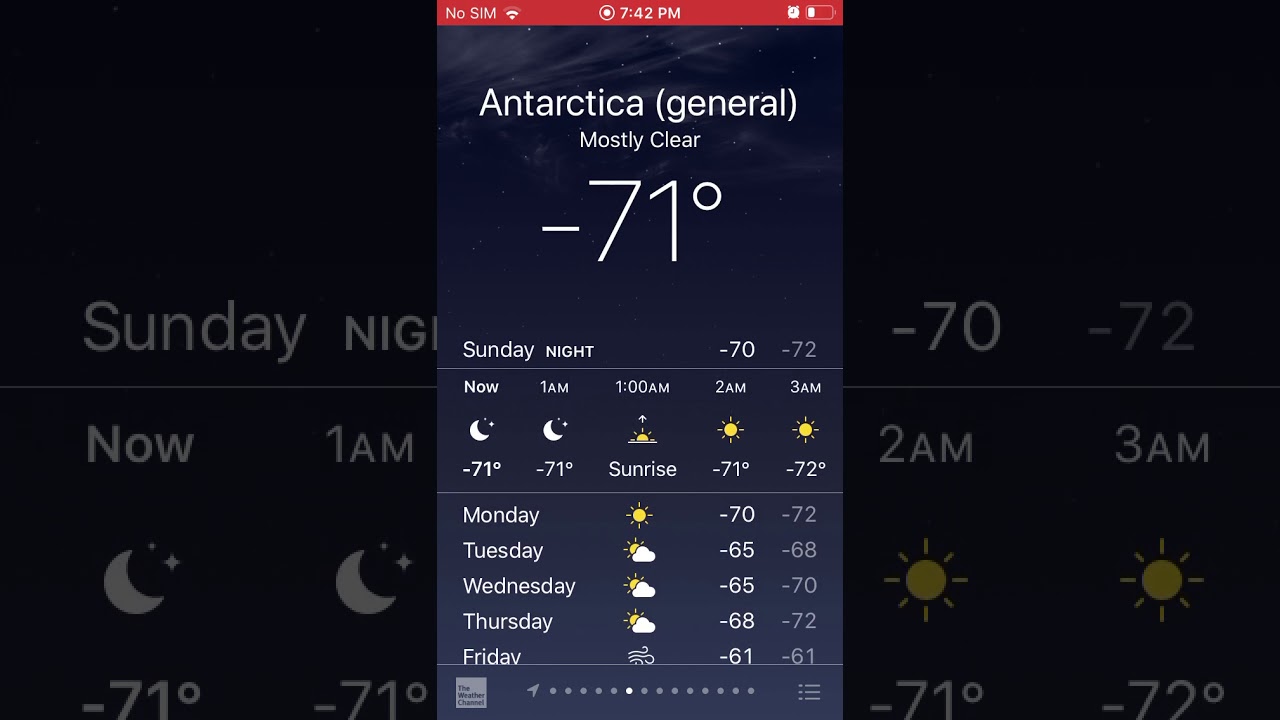The image depicts a smartphone screen with a detailed weather forecast for Antarctica. 

At the top of the screen, a red bar indicates no SIM card, no Wi-Fi connection, and no network signal, alongside a partly depleted battery icon. The current time displayed is 7:42 PM. Against a backdrop of a starry sky with scattered clouds, the text at the top reads "Antarctica" and indicates the general weather condition as "Mostly Clear." 

The temperature is shown to be a frigid -71°F. The forecast for Sunday night is detailed, with temperatures ranging from -70°F to -72°F. An icon of a half moon is present, suggesting nighttime.

Predicted temperatures for the early hours of Monday are listed as follows:
- 1:00 AM: -71°F, with the sun icon at the top indicating it is sunrise.
- 2:00 AM: -71°F, sun icon.
- 3:00 AM: -72°F, sun icon.

The extended forecast for the following days is displayed with icons that include both sun and clouds:
- Monday: -72°F daytime, -78°F nighttime.
- Tuesday: -65°F daytime, -68°F nighttime.
- Wednesday: -65°F daytime, -70°F nighttime.
- Thursday: -68°F daytime, -72°F nighttime.
- Friday: -61°F for both daytime and nighttime.

The background of the screen is largely dark, with a zoomed-in version of the weather details faintly visible, adding depth to the display. The large text highlights the substantial drop in temperature and serves as an urgent reminder of the extreme cold conditions in Antarctica.